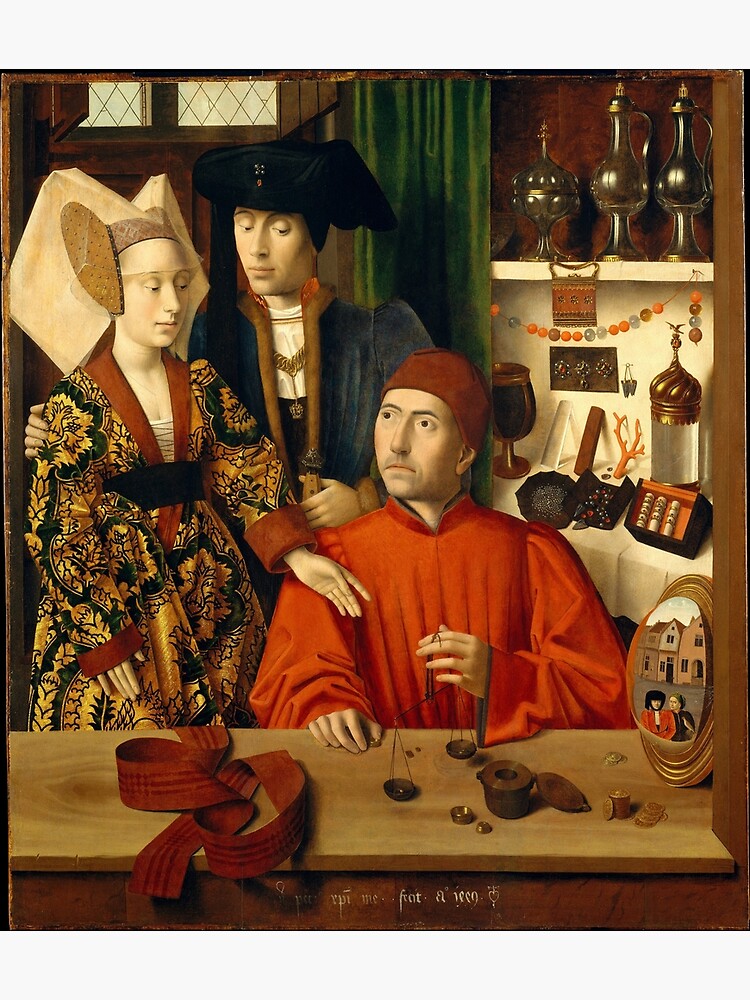This detailed painting, likely from the Renaissance period, prominently features three figures, suggesting a scene of transaction or appraisal. At its center, a man in striking red robes and a matching red hat sits at a table, meticulously holding a set of scales as if weighing or evaluating an item. His gaze is directed upwards and to his right, where a couple stands closely. The man in the couple wears a blue velvet-like robe, a white shirt, a necklace, and a black hat, while the woman beside him is adorned in an elaborate dress with gold, dark green, and orange floral patterns, highlighted by a distinctive medieval headpiece with a veil.

The background is rich with detail, showcasing a green curtain, small windows, and a shelf laden with an eclectic mix of items: large beads on a string, an embroidered purse, ornate wine vessels with spouts, a ceramic goblet, a piece of coral, and a quartz cylinder capped with gold. Additionally, a spherical mirror reflects another scene of a man and a woman against an outdoor backdrop with buildings, adding layers of intrigue to the narrative. A red ribbon lies in the foreground, enhancing the composition’s depth and color contrast.